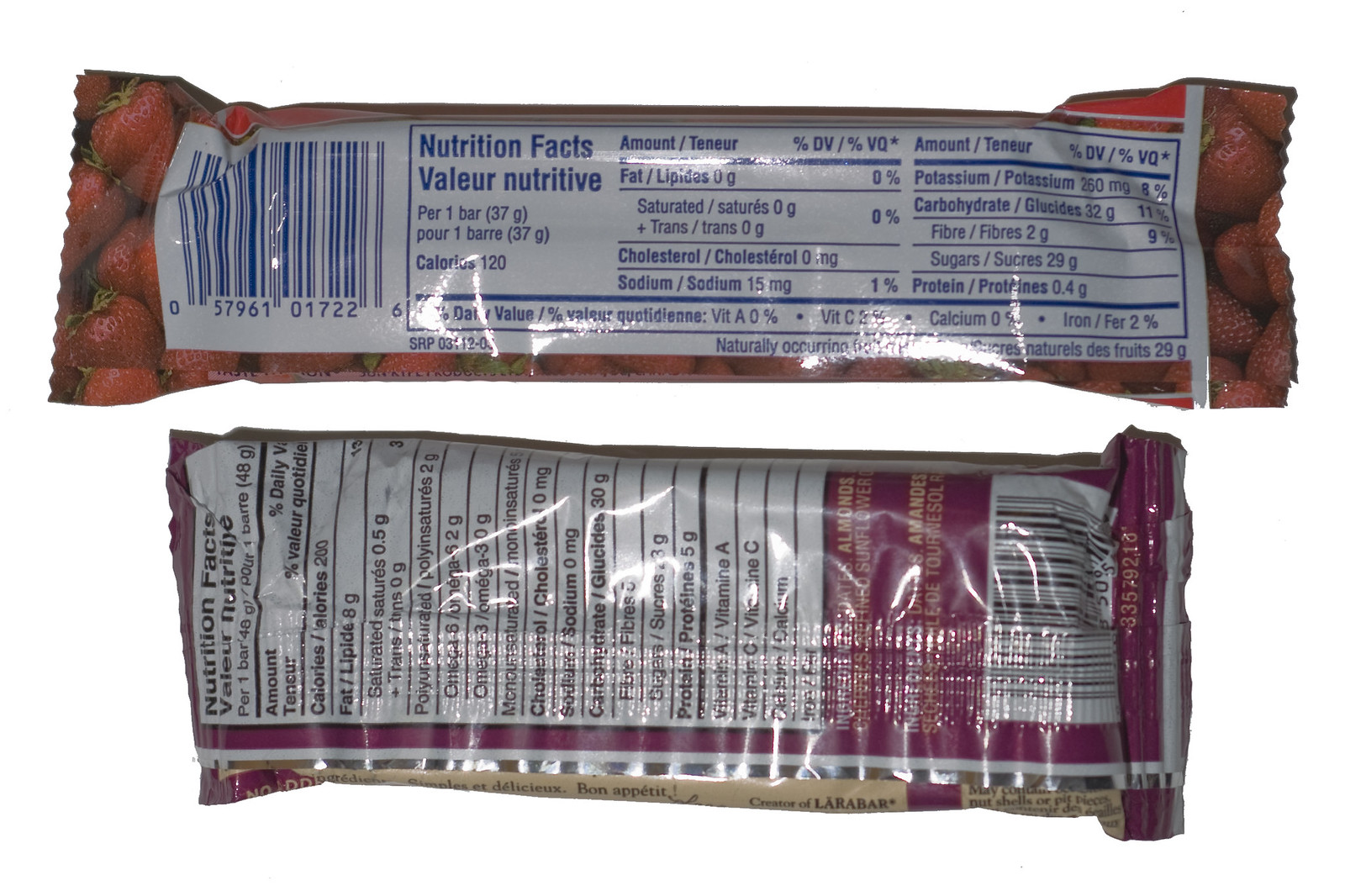The image features two snack bars, displayed with their backs visible. The first bar, positioned below, is slightly shorter and fatter. It is encased in packaging that is primarily purple with white panels, which display various nutritional values in black text. The second bar, which is placed above, is slightly longer and slimmer, wrapped in packaging with a brown background. A portion of its front is visible, revealing a striking scarlet section. Similar to the first bar, this packaging also includes nutritional information, printed in black or very dark navy lettering against a white background.